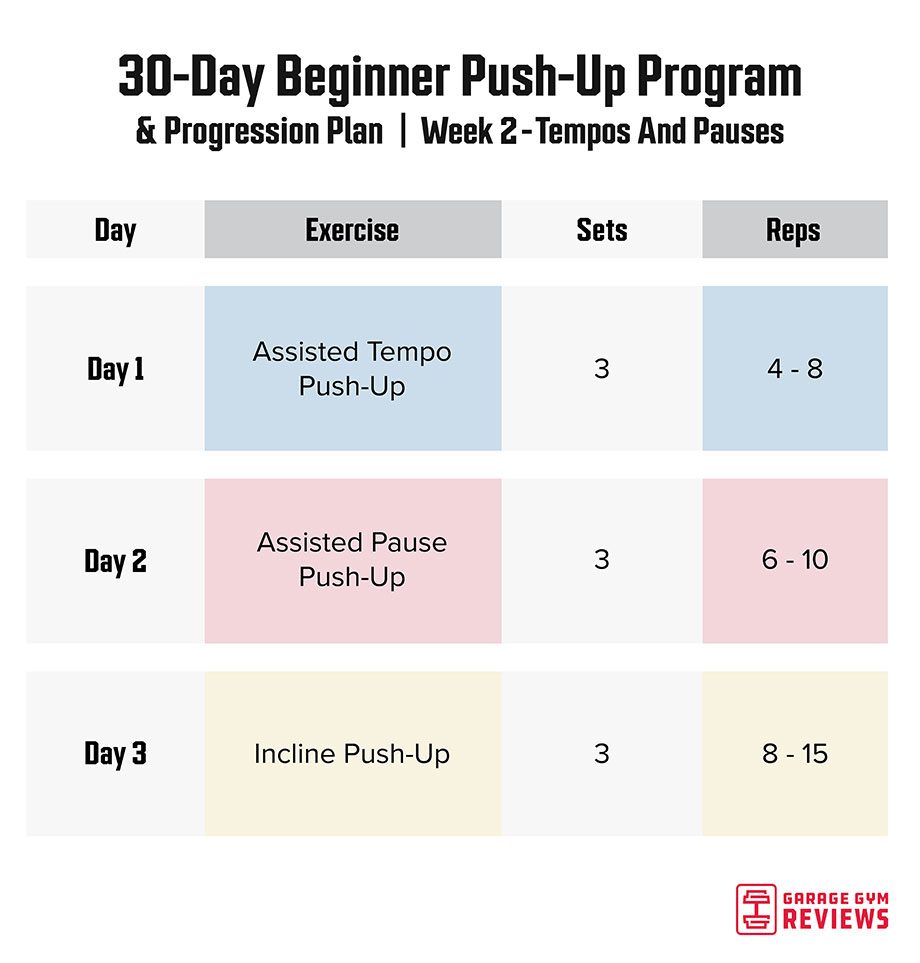The image is a detailed digital chart set against a white background, outlining a 30-Day Beginner Push-Up Program and Progression Plan. Specifically, it focuses on Week 2's "Tempos and Pauses." The chart is divided into three days, with columns labeled "Exercise," "Sets," and "Reps" across the top in gray and white boxes. 

- **Day 1**: Features an "Assisted Tempo Push-Up" with a light blue background, accompanied by "3 Sets" and "4-8 Reps" against a light gray backdrop.
- **Day 2**: Highlights an "Assisted Pause Push-Up" with a pink background, specifying "3 Sets" and "6-10 Reps."
- **Day 3**: Lists "Inclined Push-Ups" with a pale cream yellow background, indicating "3 Sets" and "8-15 Reps."

The bottom right corner of the chart features the "Garage Gym Reviews" logo in red text, accompanied by a small barbell icon inside a red box.